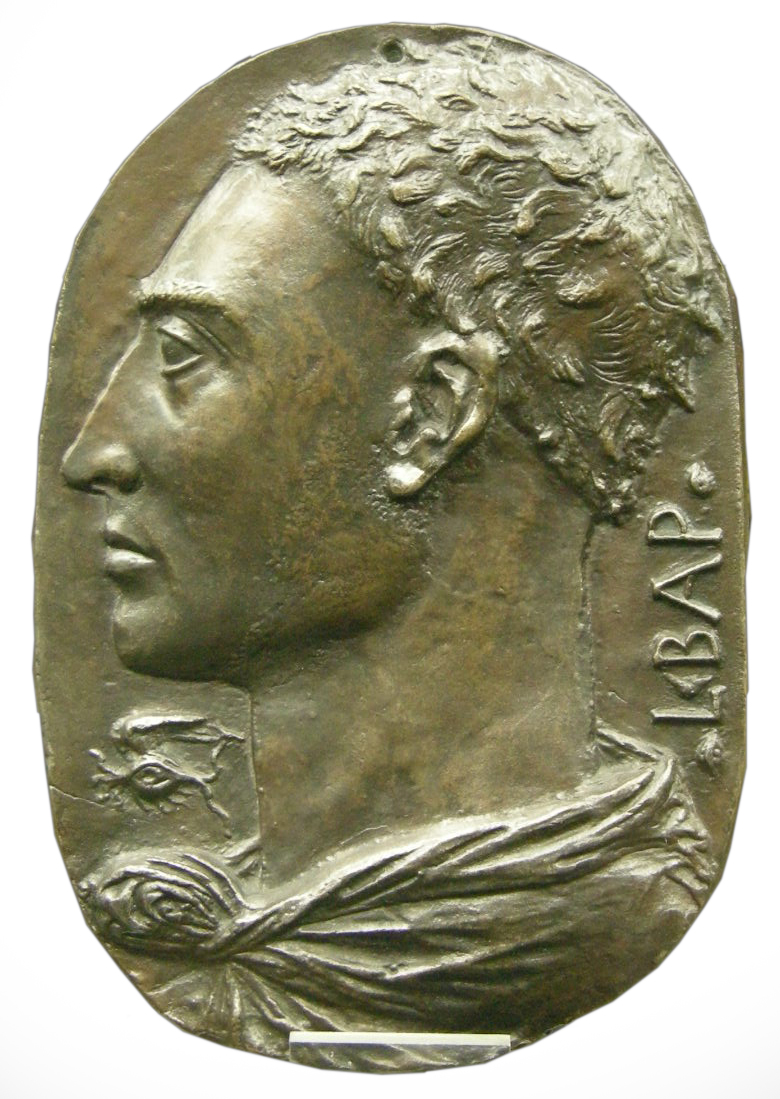The image depicts an intricately detailed carving of a man's profile, much like a relief you'd find on a bronze coin. The man is facing left, with a sharply pointed nose and a firm-set mouth. His short hair appears wavy or slightly curly, with meticulous detailing that shows the strands moving in different directions. He is adorned with a knotted scarf or cloak around his neck, with visible folds in the fabric. The material of the carving appears to be bronze or a similar metal, giving it a hard and somewhat antique surface. Along the right side of the man's profile, there are capital letters etched vertically, which read "L B A P," flanked by dots on either side. Beneath his chin, there's a hieroglyphic that resembles an eye with veins radiating outward. At the top of the image, a small hole is visible, suggesting it might be a place to pin the object, adding to its functional and decorative appeal.